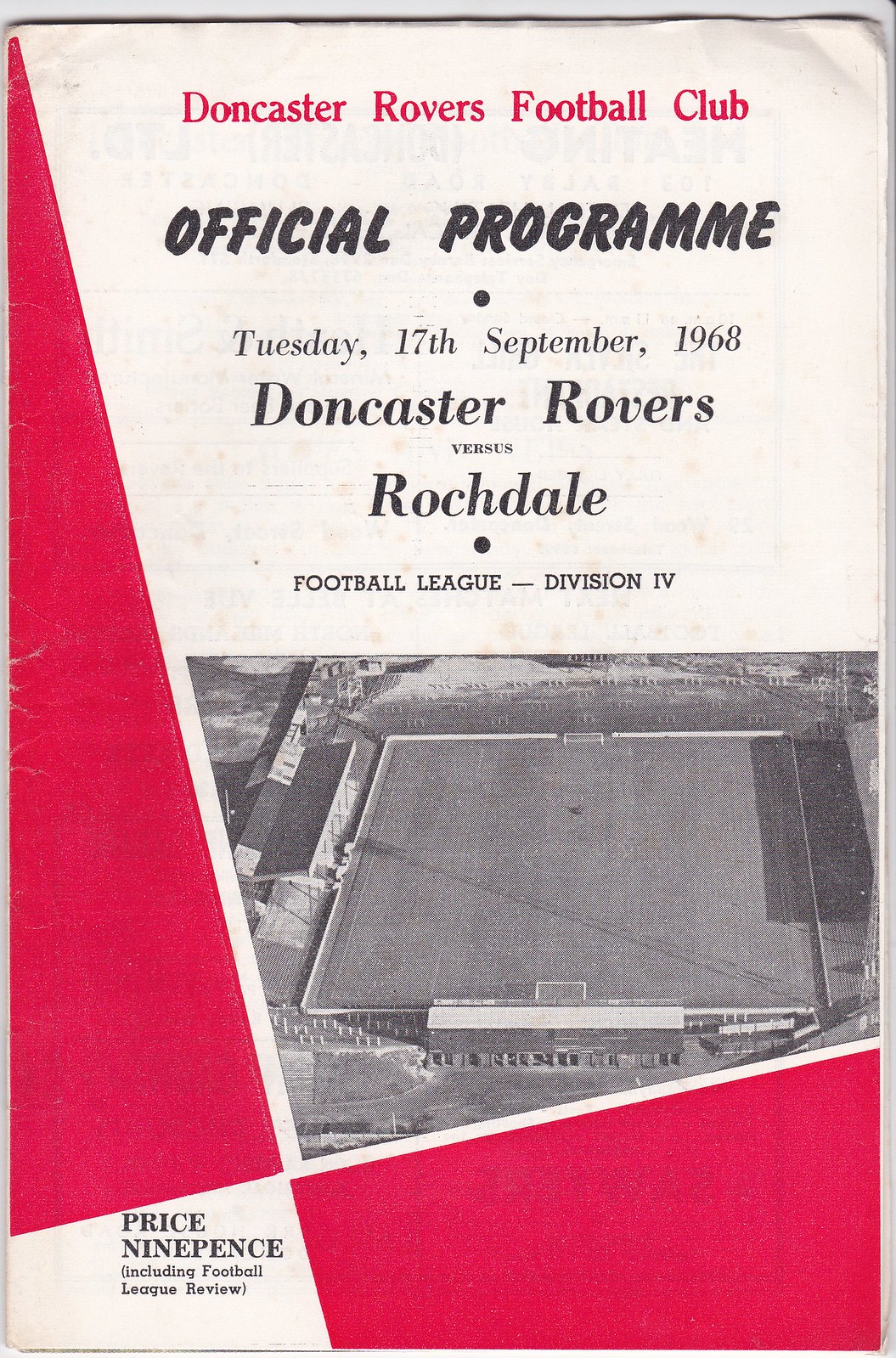This vintage pamphlet from September 17, 1968, represents an official program for a Football League Division 4 match between Doncaster Rovers and Rochdale. The background is predominantly white with striking red striping, and the text is printed in both red and black. The upper section prominently features "Doncaster Rovers Football Club" in red, followed by "Official Programme" in black. Below, details of the match date and competing teams are also in black text. Central to the pamphlet is a large black-and-white aerial photograph of an empty football stadium, situated towards the bottom. On the left side of the image, "Price 9 pence (Including Football League Review)" is written on a white panel. The layout and typography reflect the distinct design characteristics of the 1960s sports memorabilia.